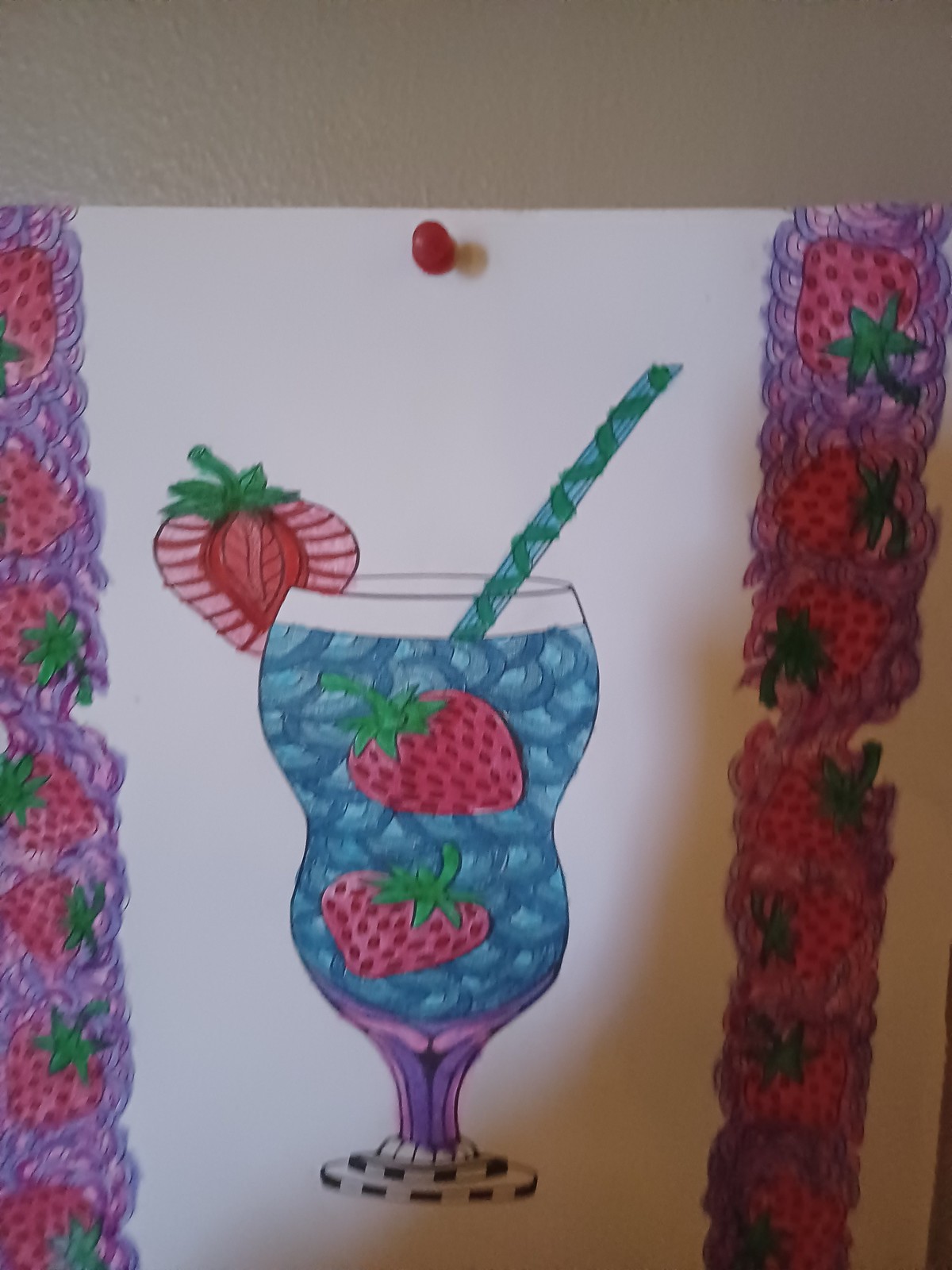The image showcases a meticulously drawn and colored drink in a curvaceous wine glass filled with a vibrant blue liquid. The beverage is characterized by numerous bubbles, each shaded dark blue on the outer rim and light blue within, adding a dynamic sense of depth. Floating within the drink are two vividly colored strawberries, distinguished by their red hue and dotted with tiny dark spots. The green stems of the strawberries peek out above the liquid, adding a touch of realism to the illustration. Emerging from the top of the glass is a blue straw adorned with diagonal green stripes, enhancing the overall whimsical appeal. The scene is framed by a patterned border of strawberries set against a circular purple backdrop, adding an artistic flourish. The artwork is presented on a white piece of paper, which is affixed to a white wall with a noticeable red tack at the top, providing a charming and casual presentation.